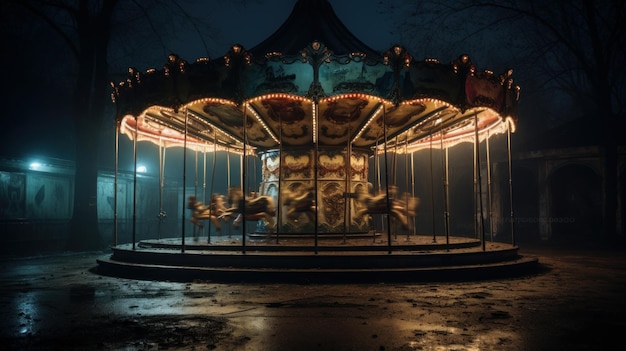The image depicts a night scene centered on an old-timey carousel with golden bars, illuminated and spinning in a seemingly abandoned setting. The wet concrete ground reflects the warm white, red, and yellow lights emanating from the strip lights around the top edge of the carousel. The horses on the carousel blur slightly, suggesting movement, adding a dynamic feel to the otherwise static environment. Surrounding the carousel, a backdrop of dimly lit buildings or walls hints at an old carnival atmosphere, with a few additional spotlights subtly illuminating the left side, contributing to the eerie, deserted ambiance. The entire scene gives a sense of both nostalgia and loneliness as the carousel, vibrant and alive, spins amidst the quiet, dark night.